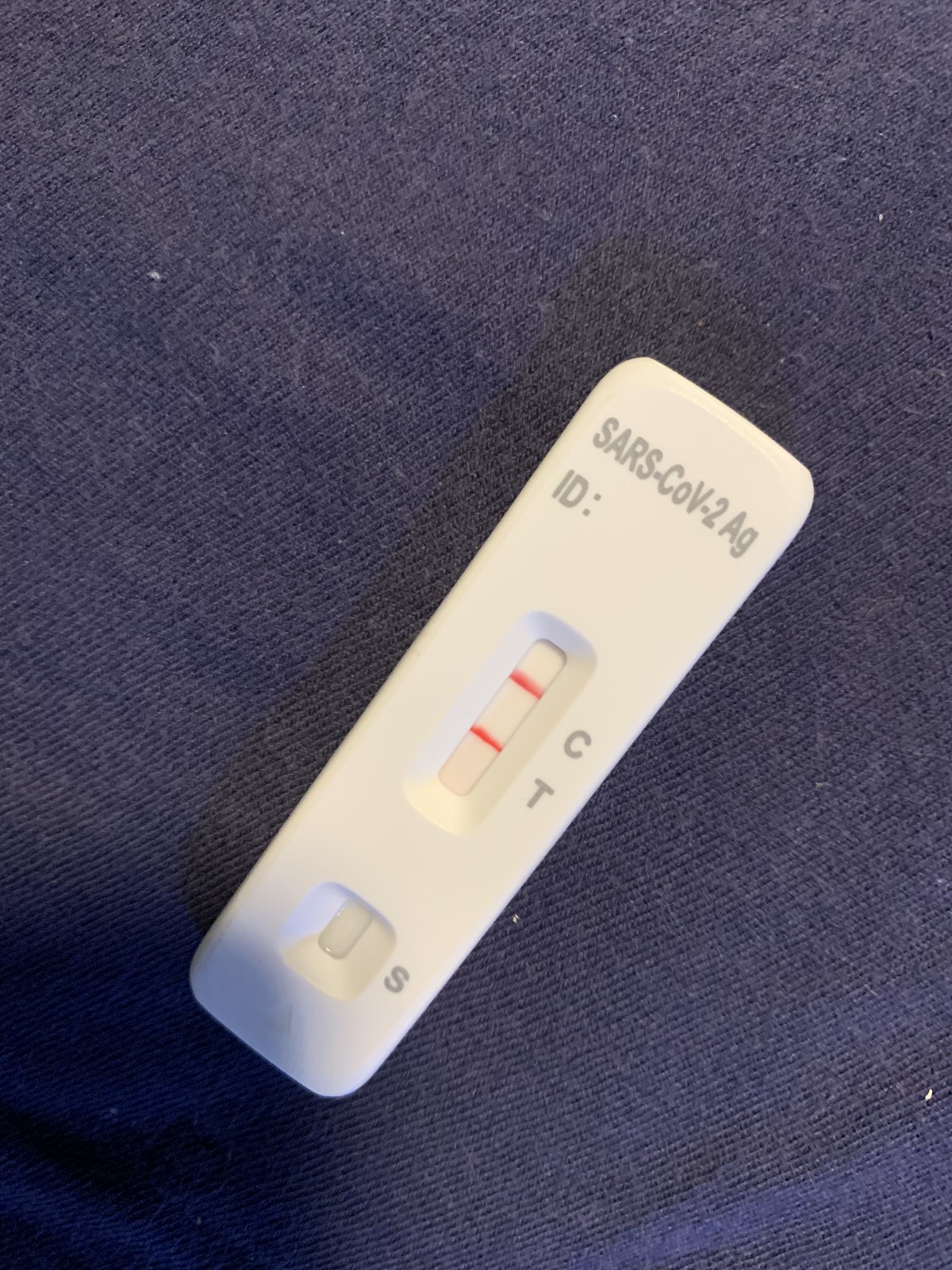A COVID-19 rapid test, indicating a positive result, is prominently displayed against a blue, ridged fabric background that could be a T-shirt, sweater, or tablecloth. At the top of the test strip, the label "SARS-CoV-2" is printed in gray, followed by an "ID:" field with a semicolon but no further identification. The test strip itself is white with two red lines—one at the "C" (control) and one at the "T" (test) markers, signifying a positive result. The casing of the test strip is also white, featuring gray letters. At the bottom of the test strip, there is a marked "S" area with a small window. The blue fabric background has noticeable ridges, adding texture to the scene, but otherwise, there is no additional context or items in the image.